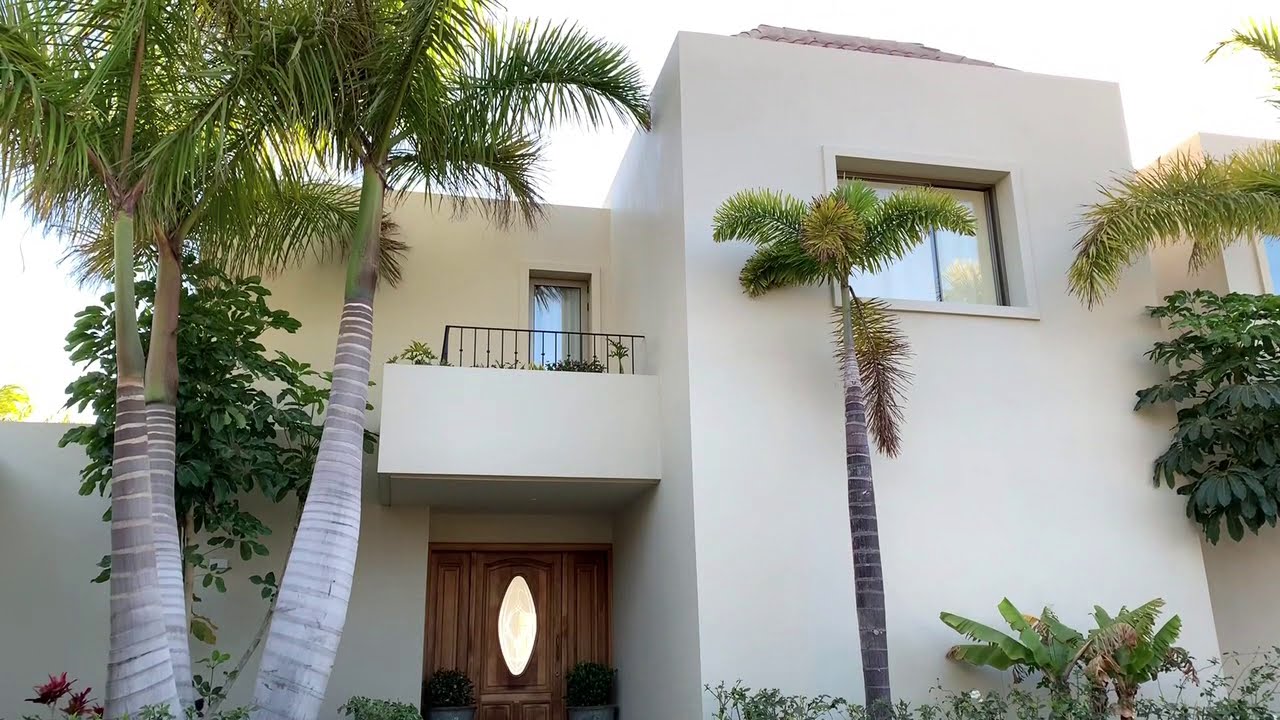The image depicts a modern, angular, two-story stucco home characterized by a blocky, rectangular architectural style. The house features a cream or white exterior complemented by a prominent wooden front door flanked by matching plants. Above the door, there is a balcony with a black railing and a glass door leading out to it. The home's minimalist design includes limited windows, specifically one on the front part near the entrance. Surrounding the house are several tall palm trees with gray trunks and lush green fronds, indicating a warm, likely southwestern, climate. The landscape also includes smaller tropical plants and green shrubbery that enhance the home's inviting front patio area. The sky in the image is clear and blue, suggesting a pleasant day.